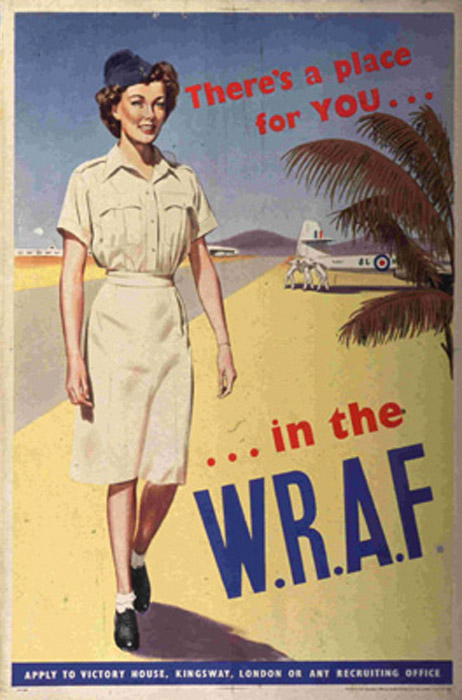This vintage advertisement for the Women's Royal Air Force (WRAF) showcases recruitment efforts, urging potential candidates to join by applying to Victory House, Kingsway, London, or any recruiting office. The image features a tropical setting, possibly evoking the climates of the Caribbean, Southeast Asia, or the Mediterranean. In the foreground, the tail of a military aircraft can be seen partially obscured by the fronds of palm trees. Rolling hills reminiscent of landscapes in Malaysia or Thailand extend into the background. A runway stretches across the scene, with a hanger visible on the far left edge, adding to the military ambiance. A woman in full WRAF uniform, complete with an official cap, beige attire, dark shoes, and ankle socks, stands prominently, embodying the era's recruitment message. This advertisement, likely from the 1940s or 1950s, effectively captures the essence of the WRAF's appeal and the historical context of its service.